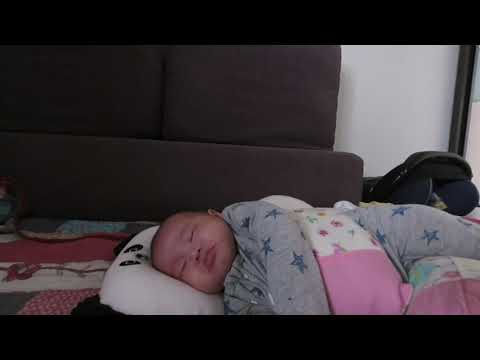The image captures a very cute, young Asian baby, possibly around one or two years old, peacefully sleeping on a carpeted floor. His head is resting on a pillow designed like a white panda bear with black ears and visible eyes. The baby is dressed in a gray pajama onesie adorned with blue stars and is partially covered by a pink blanket. A brown couch and several square boxes are visible in the background, along with white walls. The overall setting appears to be a cozy living room, as indicated by the homely furnishings and decor.